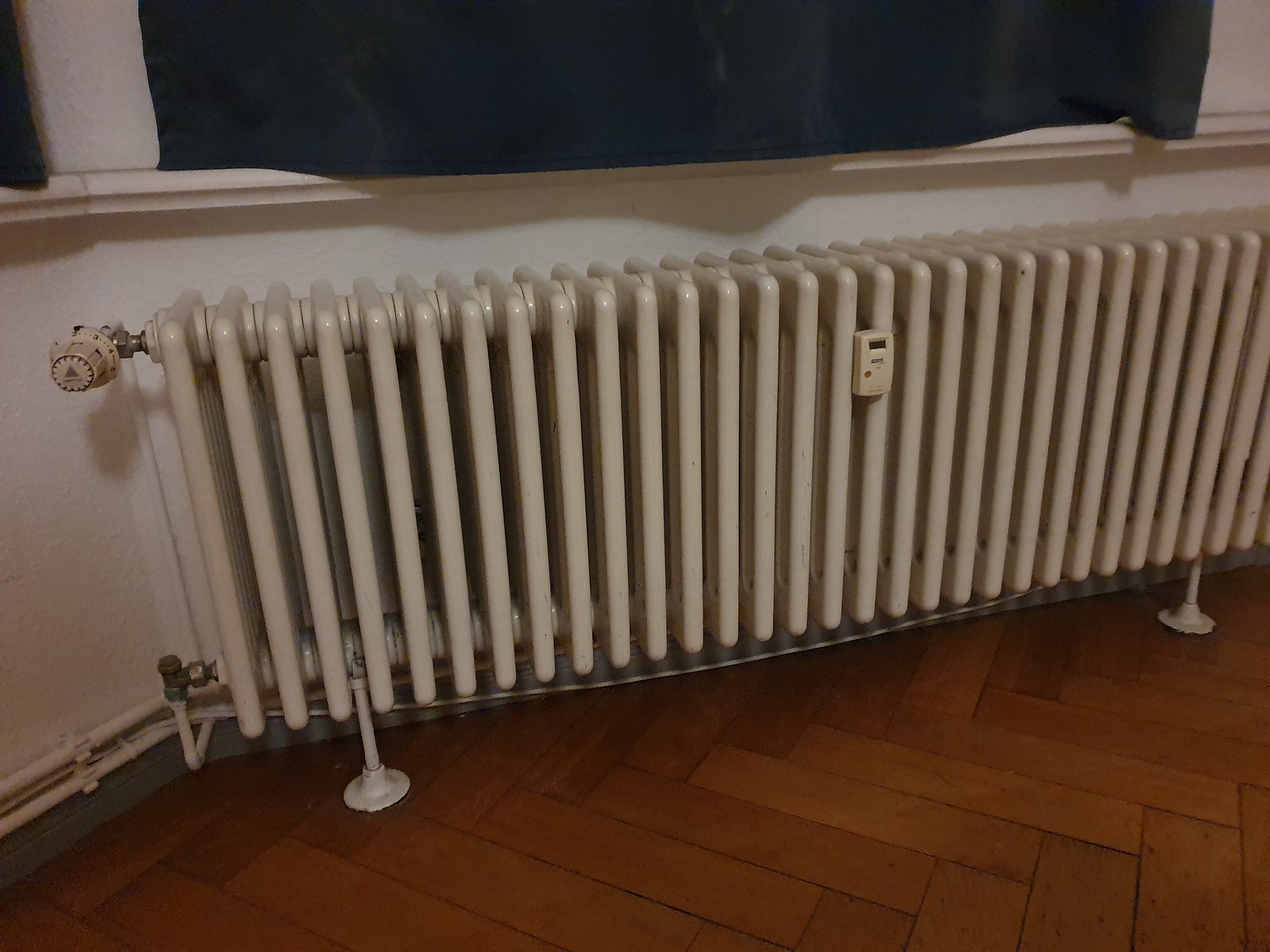The image depicts an indoor scene featuring a classic radiator set against a white wall. The radiator, a relic resembling designs from the early 1900s, is made of white metal and is connected to the building’s pipes, with metal feet anchoring it to the parquet wood floor. The floor showcases a zigzag pattern in varying shades of brown, from light tan to dark brown. Attached to the front of the radiator is a horizontal white plastic device with a small digital screen and an orange button on the left side, possibly a thermostat. The wall behind the radiator curves slightly to the left and is topped by a protruding white windowsill. Above this, black curtains frame the upper left and middle top portions of the image. Additionally, a ridge runs along the wall just below the windowsill, emphasizing the layered architectural details.